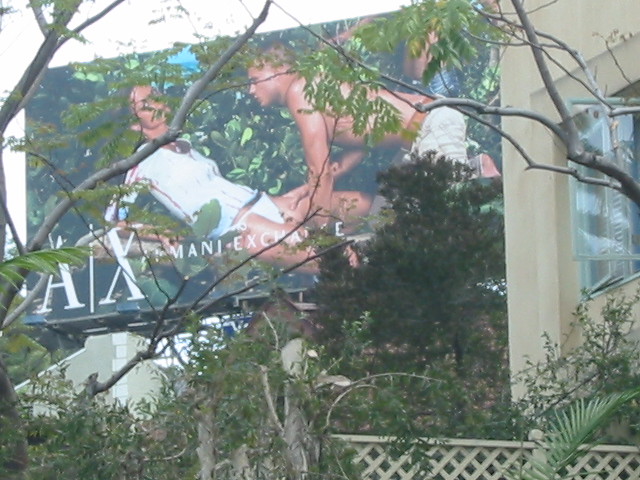The image showcases an Armani Exchange billboard partially obscured by lush greenery. The billboard prominently features the iconic 'A|X' logo and depicts two male models in an intertwined pose, suggestive of wilderness exploration, with one figure ambiguously dressed in minimal attire that appears to be a thong. In the foreground, a variety of plants, including numerous green leaves and dense branches, obscure parts of the billboard and give the scene a layered, natural feel. On the right side of the image, a tan-colored building is visible, with one window slightly ajar. Tree trunks with green foliage extend from the right edge into the middle of the composition, further adding to the image's intricate mix of urban and natural elements.